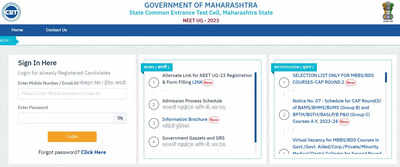A screenshot of a computer screen displaying a governmental login page. At the top of the page, there is a blue circle with the letters "CMT" inside it. Directly below, the header reads "Government of Maharashtra" in a formal font. The header section is divided into two lines: the first line features a blueprint design, and the second line has a bluish-green tint. Below this header is a section with red text, where the year "2021" is faintly visible.

On the left side of the screen, there is a sign-in section that prompts users to enter their name or email and set their password. An orange box labeled "Forgot Password" with a clickable "click here" in blue text allows users to reset their passwords. 

On the right side, there are two additional sections, each marked by a teal banner at the top. One of these sections contains the numbers 1, 2, 3, and 4, each associated with descriptive text. The adjacent section also has a similar layout with numbers listed sequentially. The overall quality of the image is blurry when zoomed in, making the text difficult to read in detail.